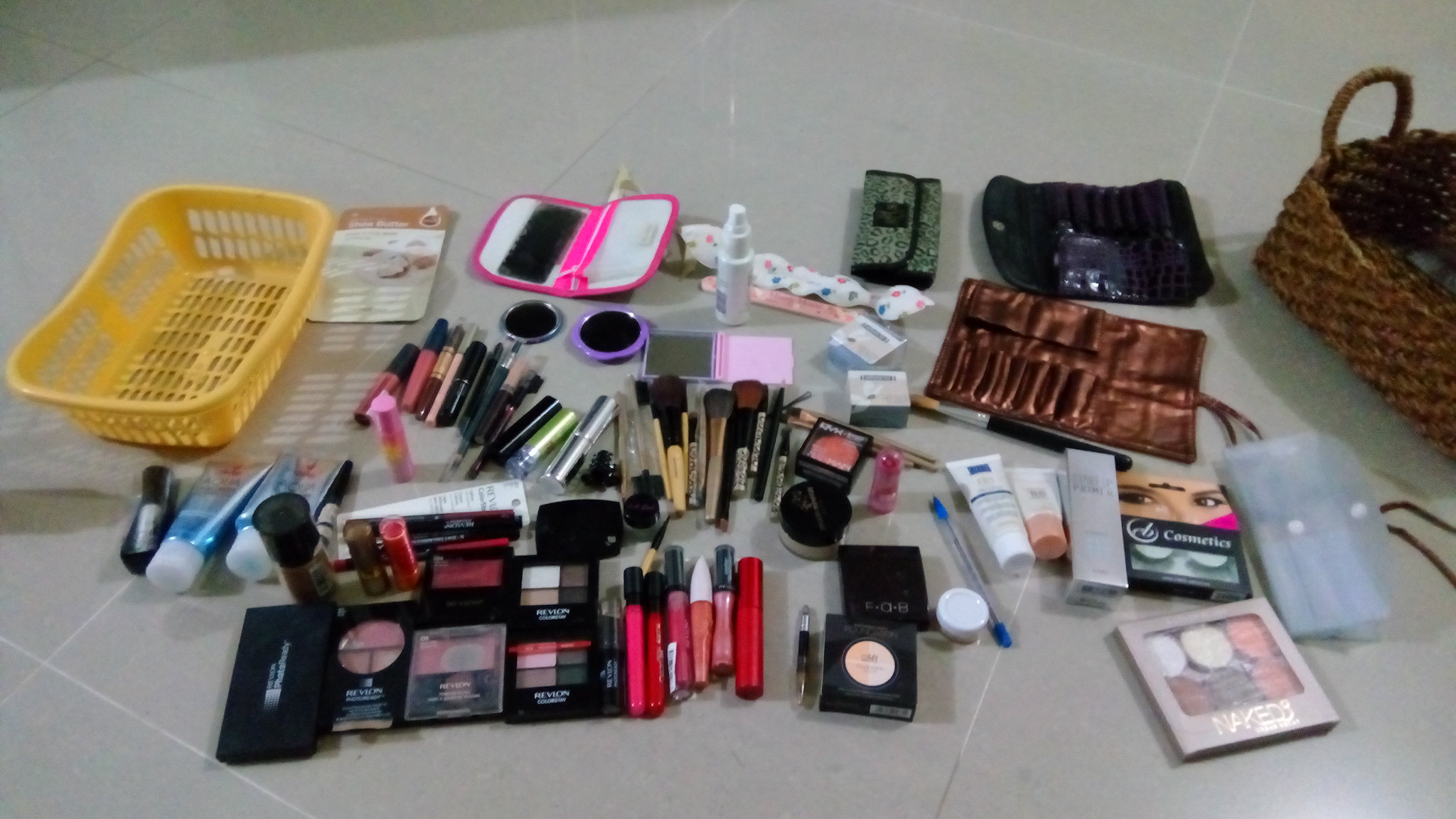This is a vibrant color photograph taken inside a store, showcasing a large floor covered in uniform, oversized white tiles. The scattered items on the floor paint a scene of disarray, focusing particularly on an assortment of makeup and accessories.

Starting from the left, there's a small, yellow basket with holes in it. Moving across the floor, the image reveals a variety of cosmetic items: a green coin purse, a slightly larger brown purse, and a blue foldable bag. In the top right portion of the photograph, a segment of a brown wicker basket is visible.

The floor is littered with numerous makeup brushes, assorted shades of concealer, different eyeliners, lipsticks in various hues, lotions, and more, creating a chaotic yet colorful spread of beauty essentials. Among the items, a noticeable blue ink pen lies amid the disarray. Additionally, there's a distinctive pink foldable mirror, currently open, revealing its reflective surfaces. Two more small round mirrors, one silver and one purple, add to the eclectic mix of scattered objects. The scene vividly captures an array of makeup products, presenting an overwhelming mix of everything one might need for makeup, all strewn across the expansive tiled floor.